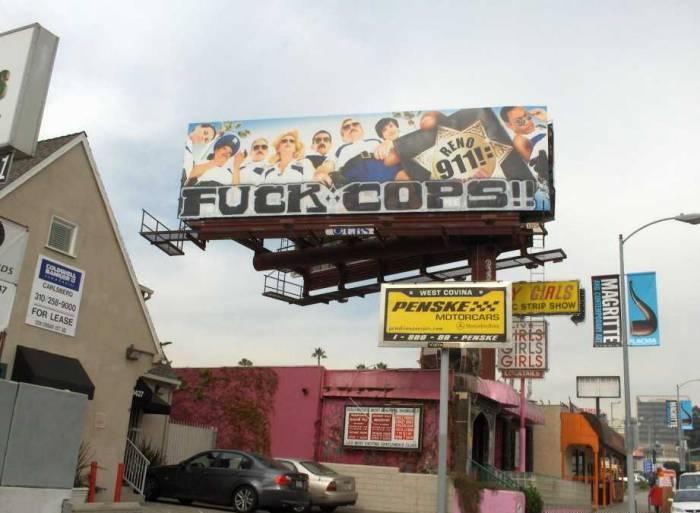This landscape-style photograph captures an urban street scene within a town. On the left side of the image, there's a home-turned-office building identifiable by a four-leaf clover sign displayed on its facade. Adjacent to this building are two parked cars. To the right, there is a prominent pink, or magenta-colored building, featuring a sign with bold letters that read "Girls, Girls, Girls." Partially obstructing the view of this building is a large yellow sign advertising "Penske Motor Cards," obscuring the complete name of the establishment, which appears to be a strip club or show venue with signage indicating something like "Girls" and "Strip Show." Dominating the composition above these buildings is a large billboard advertising the TV show "Reno 911," with a provocative message, "Fuck Cops," displayed beneath the show's title. The overall scene combines elements of commercial, residential, and entertainment properties, creating a vivid and layered urban tableau.